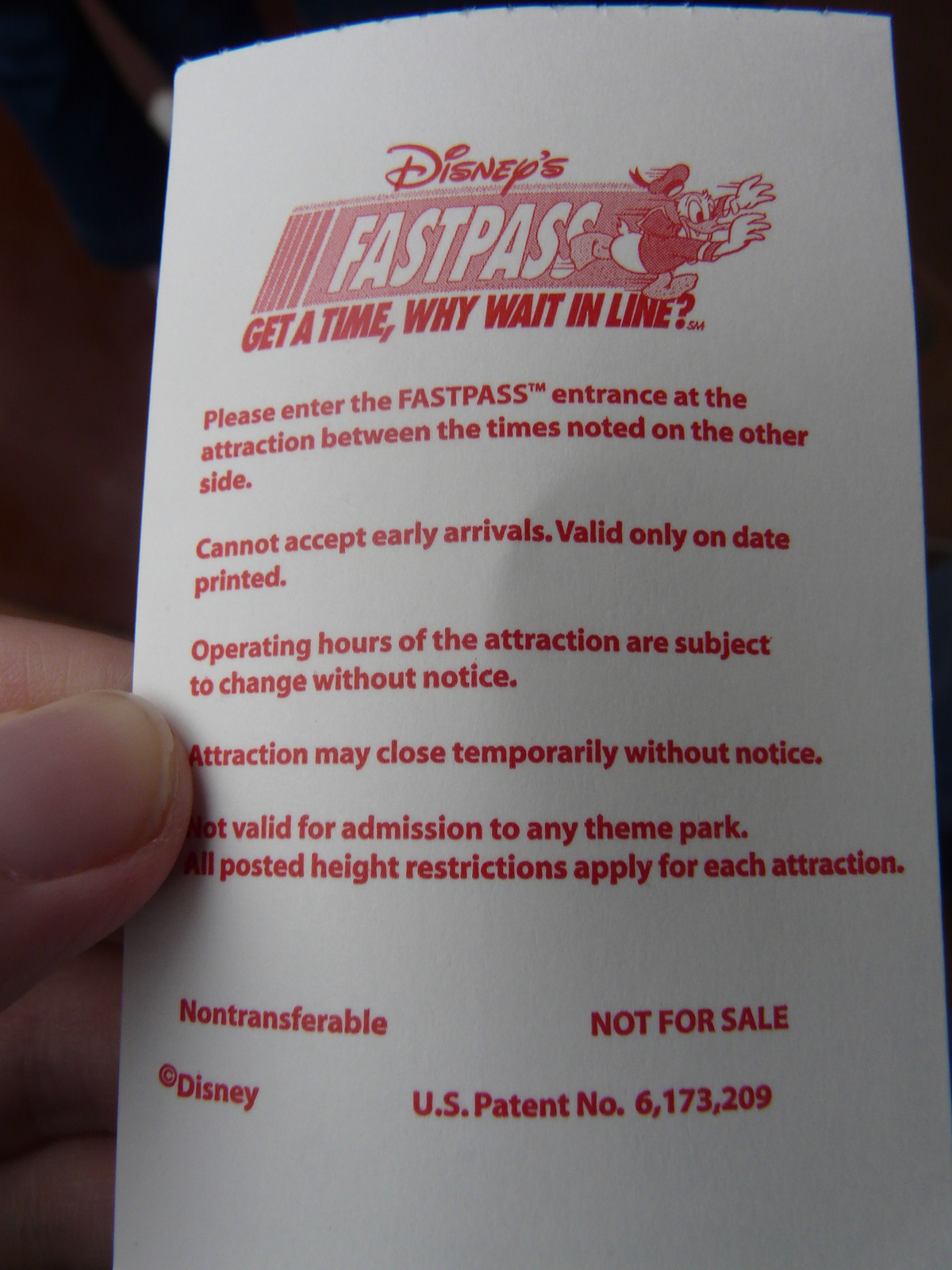The image showcases a close-up of a person holding a Disney Fastpass ticket with their thumb and a portion of their finger visible on the left side. The background is blurry, emphasizing the white ticket with red text. At the top, the ticket displays the logo "Disney's Fastpass" with an illustration of Donald Duck running with his arms up. Below the logo, it reads, "Get a time, why wait in line?" The details on the ticket instruct guests to enter the Fastpass entrance at the attraction between the times noted on the other side, with a warning that early arrivals cannot be accepted. Additional information includes that the pass is only valid on the printed date, operating hours are subject to change without notice, attractions may temporarily close without notice, it does not grant admission to any theme park, all posted height restrictions apply, and the Fastpass is non-transferable and not for sale. At the bottom, the Disney copyright and U.S. Patent number 6173209 are also visible.